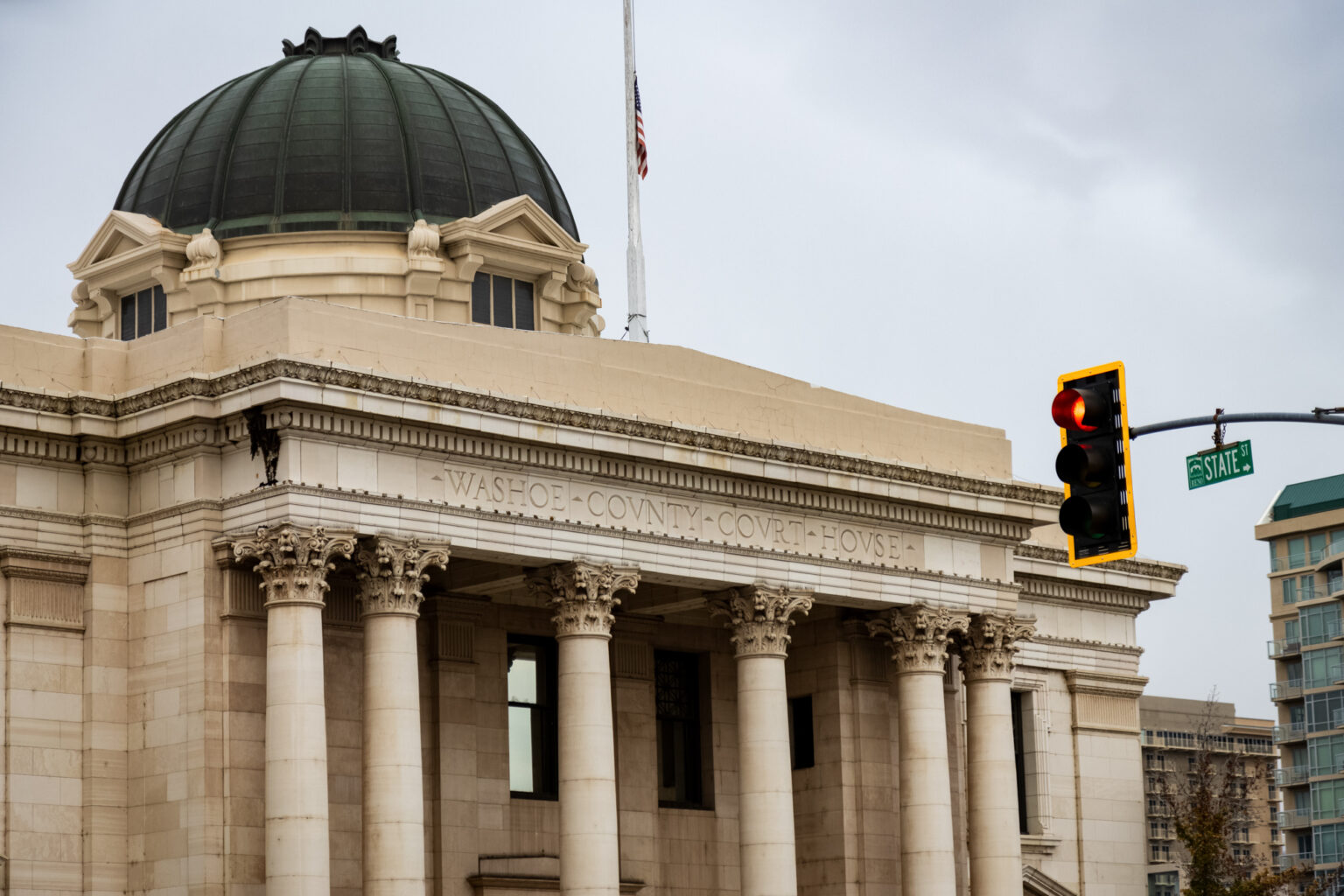This detailed color photograph captures the historic Washoe County Courthouse, constructed to emulate an old-style architectural design. The courthouse, made of large beige rectangular stone blocks, prominently displays its grand facade with six large Ionic columns supporting a gabled porch. The building is two stories tall and features a distinct green-colored metallic dome atop its flat roof, adorned with windows facing every direction. A thick, silver flagpole next to the dome proudly flies the American flag in red, white, and blue. The courthouse is central in the image, set against a dark gray, overcast sky that suggests stormy weather. A green State Street sign with white lettering is visible on a stoplight, which is turning red, positioned to the right of the courthouse. This city scene also includes other buildings to the right, along State Street, as indicated by the sign. The photograph, taken from street level in a landscape orientation, emphasizes the courthouse’s prominent architectural features and its significant placement within the urban environment.